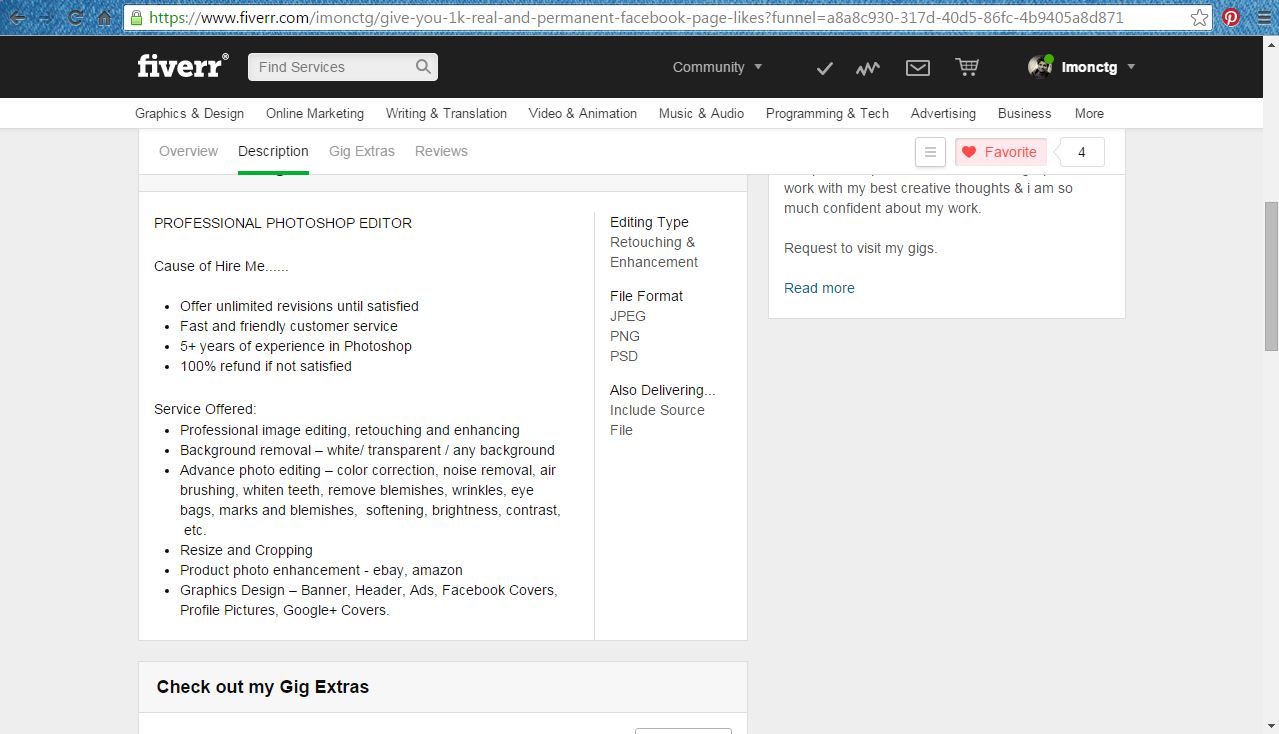The home page of a professional Photoshop editing service on the Fever website is structured with various banners, search bars, and detailed information about the editing services offered. 

At the top, there is a blue banner spanning the entire width of the page, featuring a search bar containing the web address. On the far right side of this blue banner, there is a bookmarks star, followed by a red circle with a white "P" inside, and a vertically stacked three-line menu icon.

Below the blue banner is a black rectangular banner stretching horizontally. This banner includes white text on the left that reads "Fever," adjacent to a white rectangular search bar that says "Find Services" in black text, accompanied by a magnifying glass icon. Centered within this white text, there is a "Community" tab with a drop-down menu option.

Following this is a narrower white banner with black text listing various categories, including:
- Graphics & Design
- Online Marketing
- Writing & Translation
- Video & Animation
- Music & Audio
- Programming & Tech
- Advertising
- Business
- More

Underneath this category banner are tabs for different sections: "Overview," "Description" (highlighted in green), "Gig Extras," and "Reviews." On the far right of this tab line is a square with three lines, followed by a pink rectangle with red text and a red heart that indicates "Favorite."

The main body of the page begins with a large white square on the left, showcasing black text that reads "Professional Photoshop Editor." Below this headline, there are key points about the service:
- "Cause of Hire Me."
- "Offer unlimited revisions until satisfied."
- "Fast and friendly customer service."
- "Five plus years of experience in Photoshop."
- "100% refund if not satisfied."

The service offerings are listed in detail:
- Professional image editing, retouching, and enhancing.
- Background removal (white, transparent, or any background).
- Advanced photo editing including color correction, noise removal, airbrushing.
- Cosmetic edits such as teeth whitening, blemish, wrinkle, and eye bag removal, softening, brightness, and contrast adjustments.
- Resize and cropping options.
- Product photo enhancement suitable for eBay and Amazon.
- Graphics design for banners, headers, ads, Facebook covers, profile pictures, and Google Plus covers.

To the right of these service details, the page lists:
- Editing type: Retouching and Enhancement.
- File format options: JPEG, PNG, PSD, with source files included upon delivery.

Finally, there is a personal note from the service provider stating their dedication and confidence in their work, encouraging visitors to explore more of their gigs with a "Read More" link.